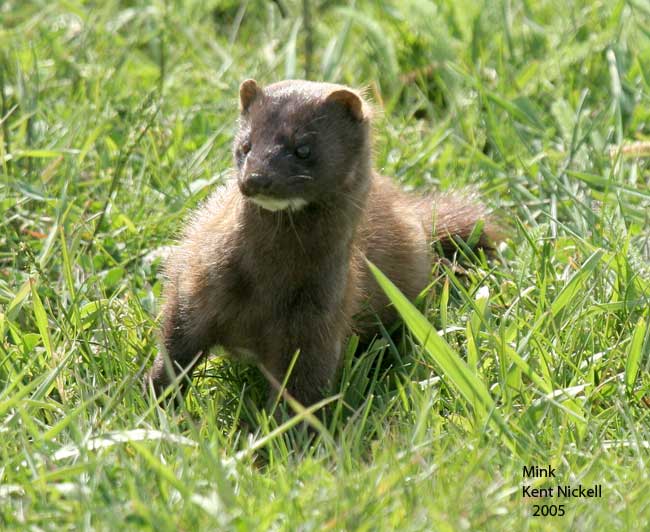The photograph features a brown mink, a long-bodied creature with a white scruff under its chin, black nose, and small rounded ears. Its two round, black eyes are fixed intently on something off-screen, giving it a very alert pose. The mink is captured at eye level amidst a field of lush, green grass, which surrounds it completely. It stands on all four paws, with its body slightly facing forward and to the left, and a tail that extends to the right. Multiple thin whiskers are visible around its snout. In the lower right corner of the image, there's black text that reads "Mink, Kent Nickel, 2005."